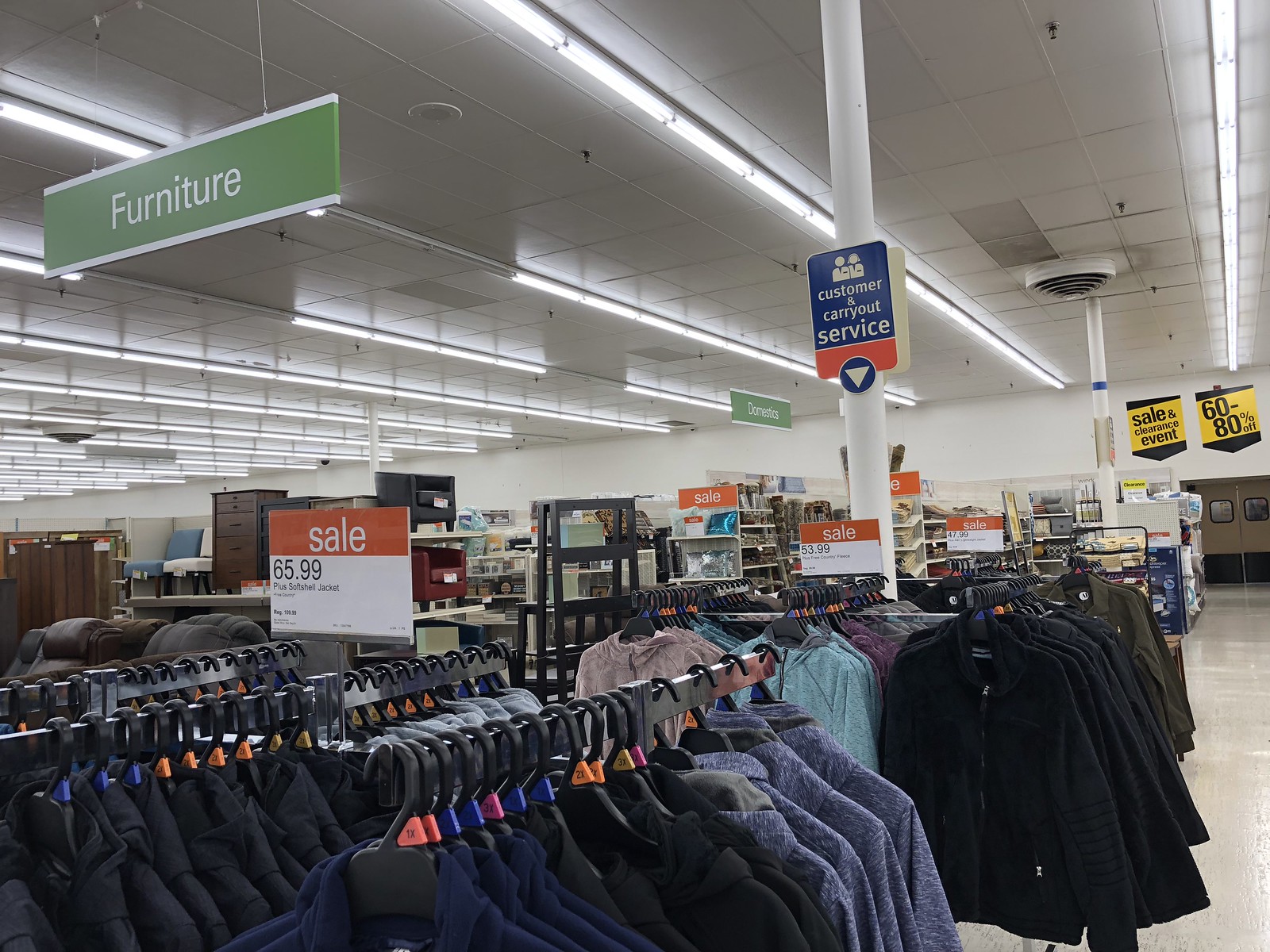The image captures the bustling interior of a multi-use general store. In the foreground, there is a display of men's clothing, featuring an array of sweaters and jackets neatly hung on black hangers, which are mounted on sturdy steel racks. Above this section, a prominent sign advertises a sale with prices starting at $65.99. 

Moving upwards towards the ceiling, a large sign with white lettering on a light avocado olive background directs customers to the furniture section. Further back in the store, another sign informs shoppers about the "Customer and Carry Out Service." 

In the distant background, two bright yellow signs catch the eye, announcing a significant sales and clearance event with discounts ranging from 60 to 80 percent off. The image effectively portrays the diverse offerings and organized layout of the general store, emphasizing the various sections and promotional deals available to customers.